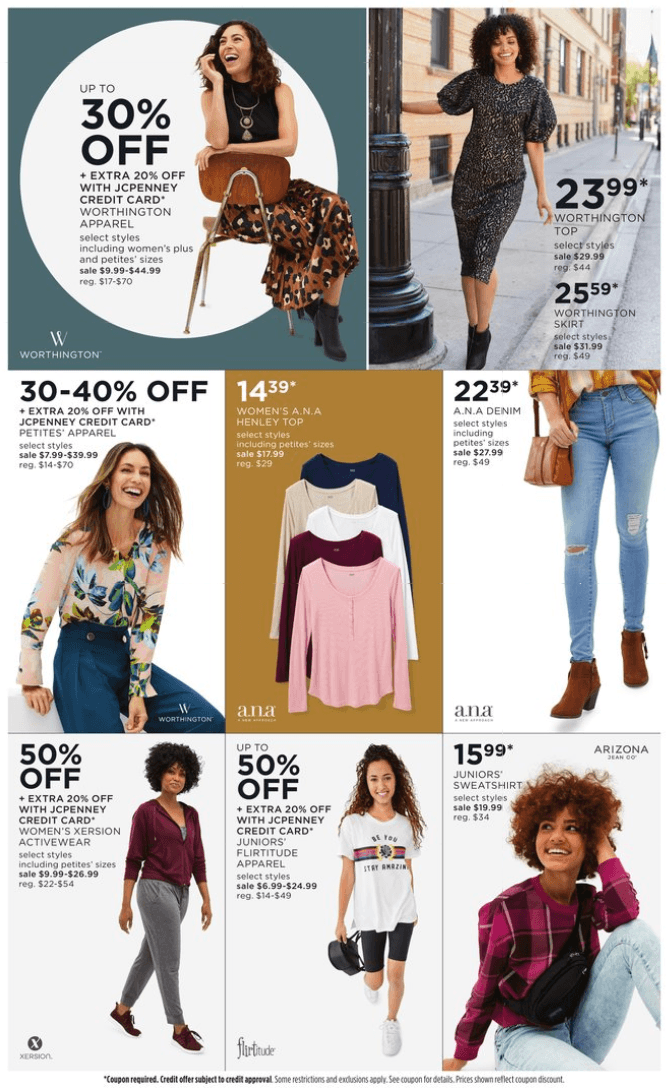This image appears to be a screenshot from a multi-brand clothing advertisement, possibly sourced from a magazine. The layout is visually organized, showcasing different apparel items with price tags and offers. 

In the top left-hand corner, a white circle highlights a promotional offer stating "Up to 30% off." 

To its right, there's a picture of a woman seated on a brown chair, dressed in an elegant dress, with a warm smile on her face. 

Adjacent to her, another woman is seen leaning against a lamppost, donning a sparkling black dress priced at £23.99. 

Below these images, a close-up shot of light blue skinny jeans is prominently featured, tagged at £22.39. 

To the right of the jeans, a collection of four long-sleeve henley tops is laid out against a mustard yellow background, each priced at £14.39. 

Adjacent to this section, a woman wearing a blouse, with a bright smile, is advertised, noting a discount range of 30-40% off. 

At the bottom, a series of three images shows girls walking, dressed in various outfits comprising jeans, shorts, or leggings paired with different blouses.

Overall, the advertisement effectively highlights a range of stylish women’s clothing options available at discounted prices, catering to different tastes and preferences.